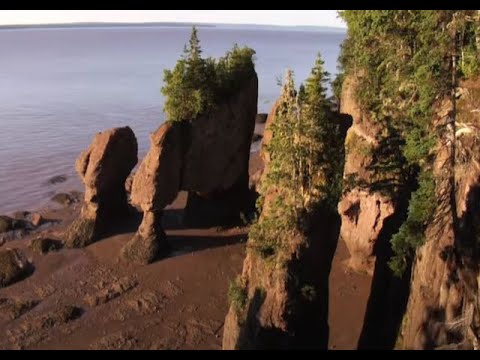This vibrant aerial photograph, presented in landscape mode with thin black borders at the top and bottom, captures a dramatic coastal scene. Central to the image are tall, jagged rock columns and cliffs along the coastline, their steep and sharp drops partially covered in lush greenery, including coniferous trees and various shrubs. The brownish, mud-colored earth stretches out beneath these rocky formations, creating a stark contrast to the smooth blue sea visible in the top left corner of the photo. The ocean appears calm, reflecting the light from the whitish daytime sky seen in the uppermost part of the image. Scattered rocks jut out from the water’s edge, hinting at the rugged nature of the shoreline. In the distance, another strip of coastline suggests the potential setting of a bay, enhancing the depth and realism of this picturesque seascape.